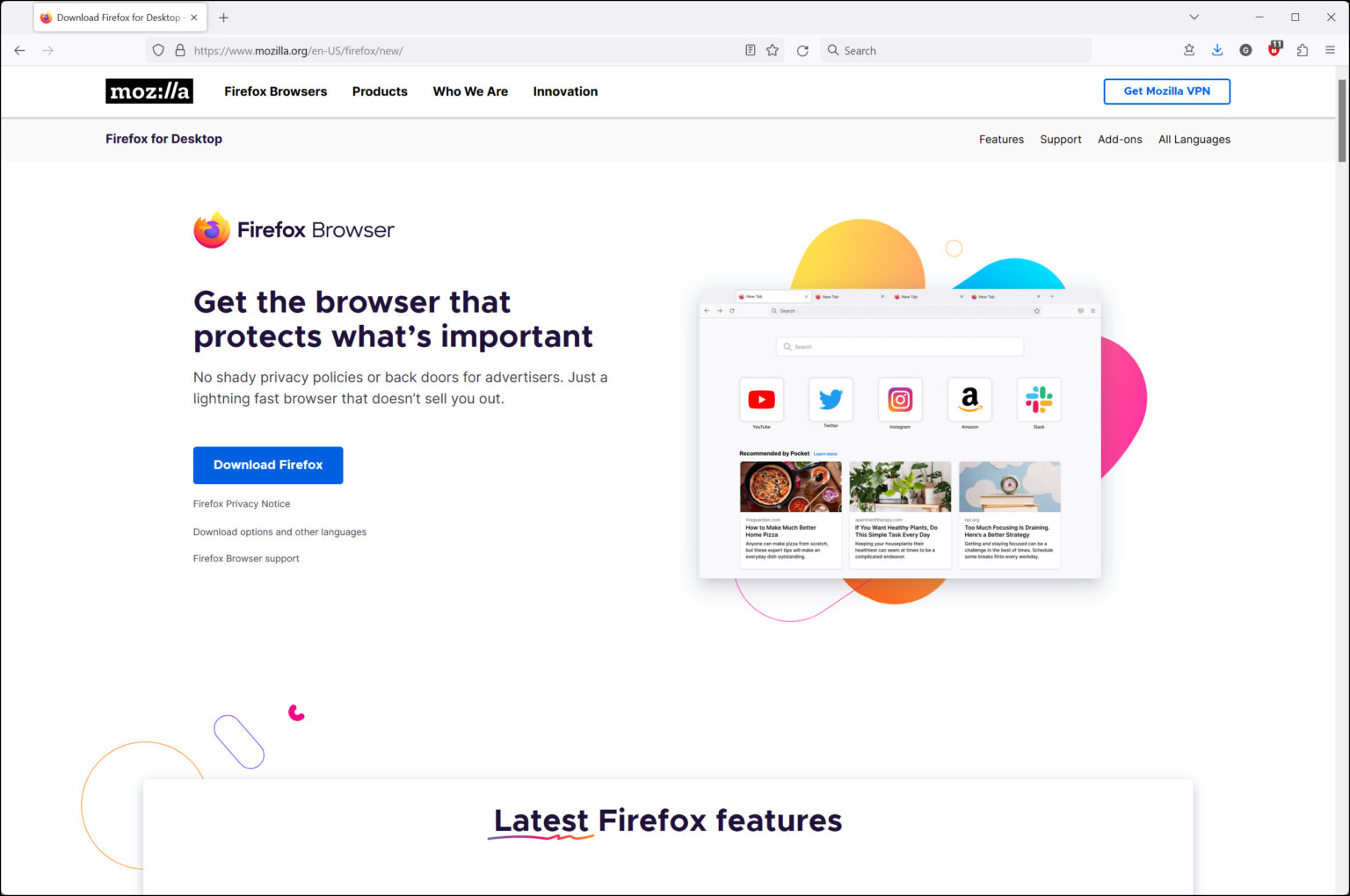Screenshot of the Firefox Browser Download Page:

At the top of the page is a navigation bar with a black rectangle featuring white text that reads "Mozilla." Adjacent to it, in black text on a white background, are the options: "Firefox Browsers," "Products," "Who We Are," and "Innovation." Below this is another navigation bar in a very pale gray, listing: "Feedback for Desktop," "Features," "Support," "Add-ons," and "Languages." 

The main content area has a white background with black text. Positioned at the top left is the Firefox logo. Next to it, bold text reads "Firefox Browser." On the right side of the page, there's an image of the Firefox browser. Below the Firefox logo, a headline proclaims, "Get the browser that protects what's important."

At the bottom of the page, the footer message highlights "Latest Firefox Features."